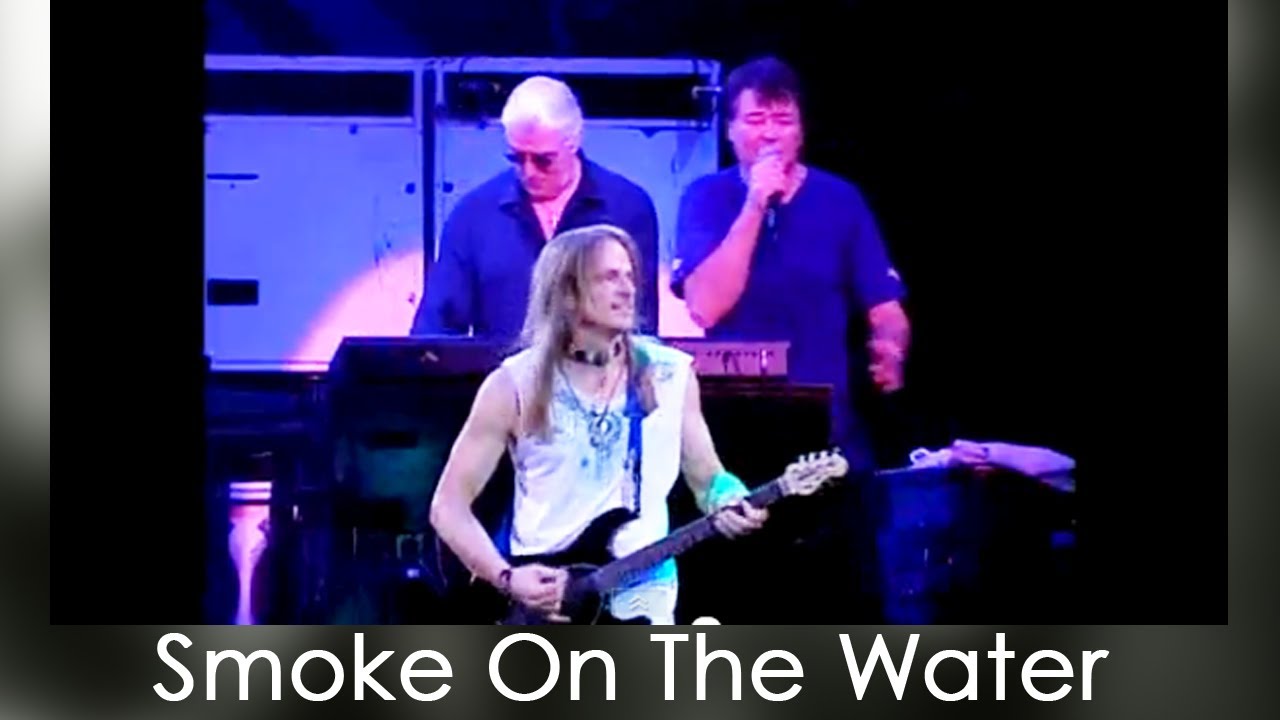The photoshopped image portrays a group of three musicians on stage, captured in the midst of a live performance. The focal point is the frontman with long blondish-brown hair, reminiscent of a young Ted Nugent. He confidently plays a black electric guitar while sporting a white top. Behind him, two other band members contribute to the scene; one dressed in a blue shirt passionately sings into a microphone, while the other, also in blue, plays the keyboard. The background is dark, suggesting a nighttime stage setting. At the bottom of the image, white text reads "Smoke on the Water," indicating that they are performing the iconic song by Deep Purple, although it should be noted that Ted Nugent is not typically associated with this track.